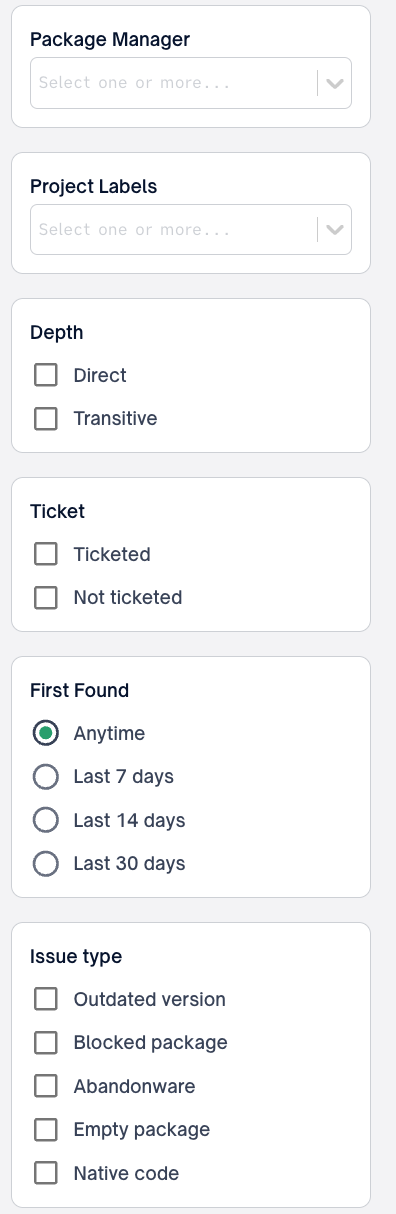This is a detailed screenshot of a graphical user interface, set against a light gray background and predominantly featuring white and gray elements. At the top, a white rectangular section is bordered in light gray, containing the bolded black text "Package Manager" on the left.

Below this header, another gray-outlined rectangle holds a prompt in very light gray text: "Select One or More," adjacent to a vertical gray line. To the right of this line is a downward-pointing arrow resembling a 'V'.

Further down, a similar white rectangle titles a section with the bolded black text "Project Labels." Within this section is another search bar with the same "Select One or More" instruction.

Proceeding downward, another larger white rectangle features various settings. In the upper left-hand corner, the bolded black text "Depth" labels the section. Here, two boxes outlined in gray represent options, with the text "Direct" to the right of the first box and "Transitive" to the right of the second box.

Continuing within the same rectangle, the label "Ticket" appears in bolded black. Below this, two more gray-outlined boxes are displayed, the first marked "Ticketed" and the second "Not Ticketed."

The next segment involves temporal filtering, indicated by the bolded black text "First found." Below this, vertically-aligned gray-outlined ovals list time ranges: "Any Time," "Last 7 Days," "Last 14 Days," and "Last 30 Days." The oval corresponding to "Any Time" contains a filled green circle, signifying selection.

The last section, labeled "Issue Type" in bolded black, presents a set of options represented by squares. These options include "Outdated Version," "Blocked Package," "Abandoned Ware," "Empty Package," and "Native Code."

This comprehensive layout allows for extensive filtering and selection within the interface.